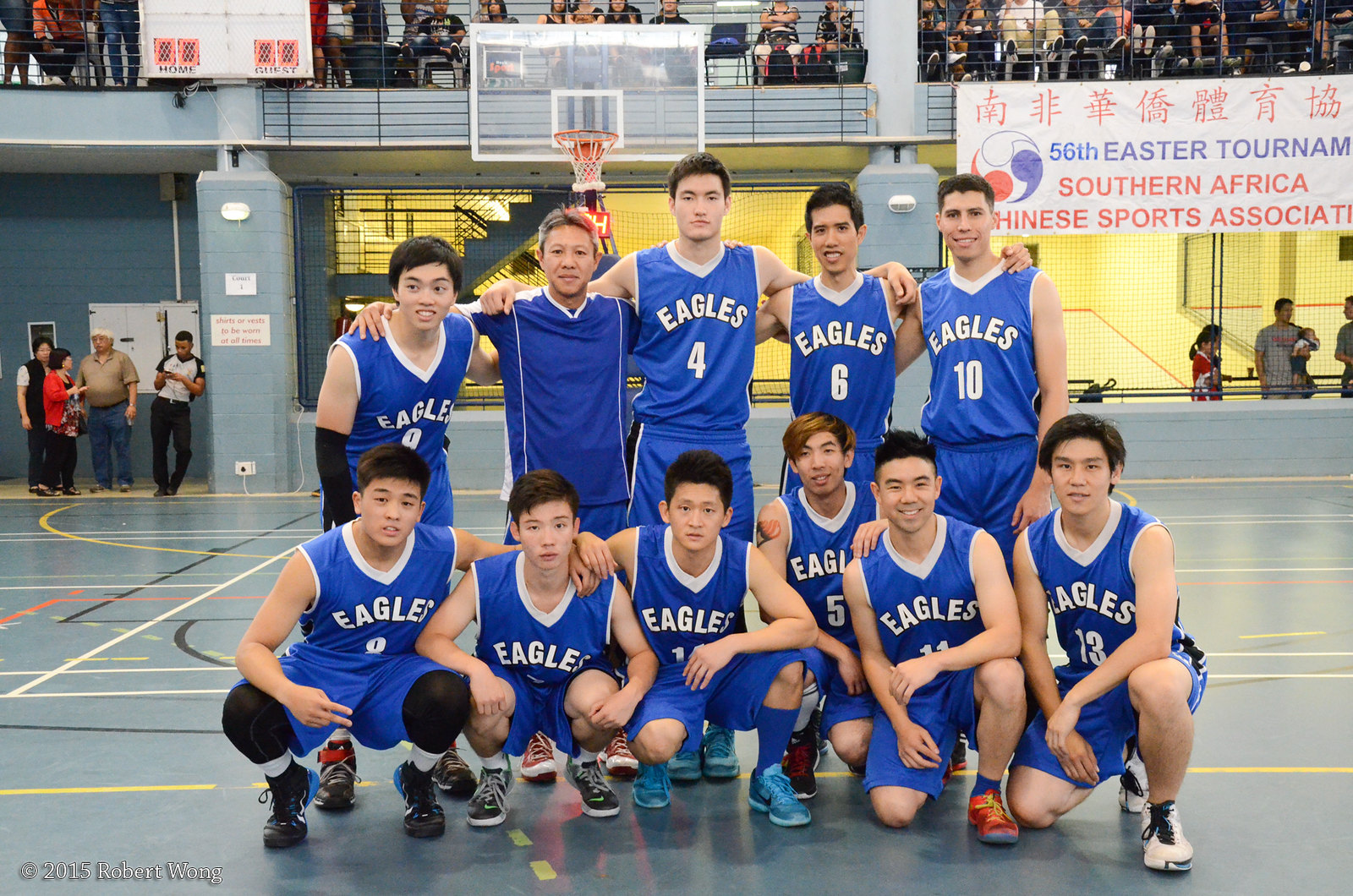The image showcases an Asian basketball team of 11 players in a gym, posing for a team photo. They are wearing blue sleeveless tunics with the team name "Eagles" in white font, and matching blue shorts, without a standardized sneaker or sock uniform. The players are arranged in a triangular formation, with the front row kneeling or squatting and the back row standing tallest in the center. Behind the team, there are tall basketball hoops and the gym floor features aqua-teal color with yellow, white, black, and red lines marking different boundaries. In the background, a white banner reads "56th Eastern Tournament, Southern Africa, Chinese Sports Association." The gym has gray pillars, gray bleachers with some spectators, and a red and blue yin-yang style sign. Several adults, some leaning against a pillar and others behind a table under the banner, are visible in the background.